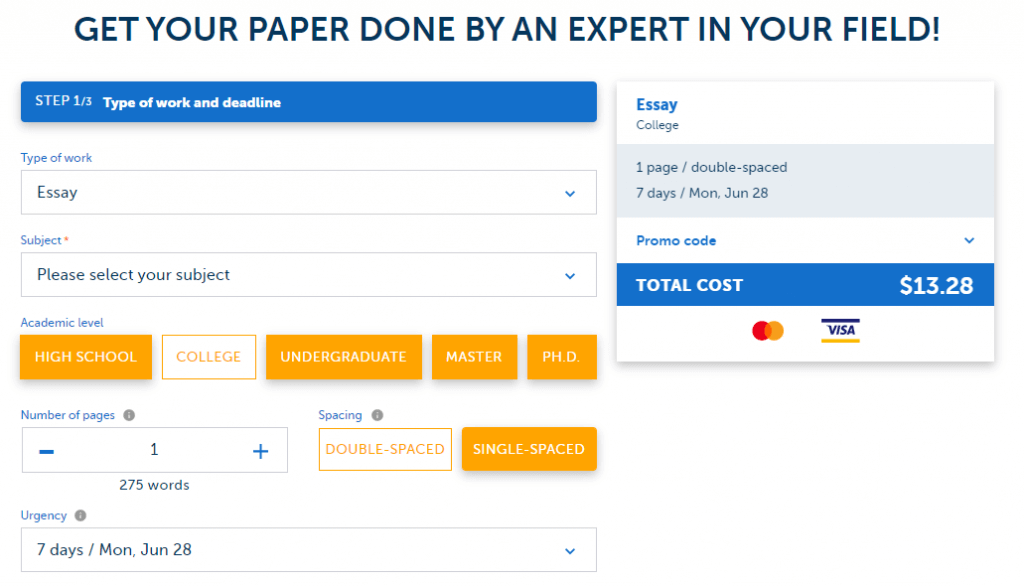At the top of the stark white webpage, bold black letters prominently display the headline: "Get your paper done by an expert in your field." Below, on the left-hand corner, inside a blue square with white lettering, it states "Step one of three: Type of work and deadline." This section requires users to choose the type of work, like "essay," and provides details about the deadline, specifying "seven days" with a due date of "Monday, June 28th."

On the right-hand corner, further specifics are given: "Essay, College, One page, Double spaced, Seven days, Monday, June 28th." The page also includes a "Promo code" field and displays the "Total cost: $13.28" alongside logos for MasterCard and Visa to indicate accepted payment methods.

Adjacent to these details, the page asks for the type of work again, listing "Essay" as an example, followed by a prompt to select the subject. It also provides options for the academic level, ranging from high school to PhD. The user can specify the number of pages, the spacing preference (double or single spaced), with an indication that each page is approximately 275 words.

Throughout the page, color accents in shades of orange, blue, white, and dark blue highlight various sections, adding visual interest and guiding the user through the form. The form concludes with a request for the urgency of the assignment, reiterating the seven-day deadline of "Monday, June 28th."